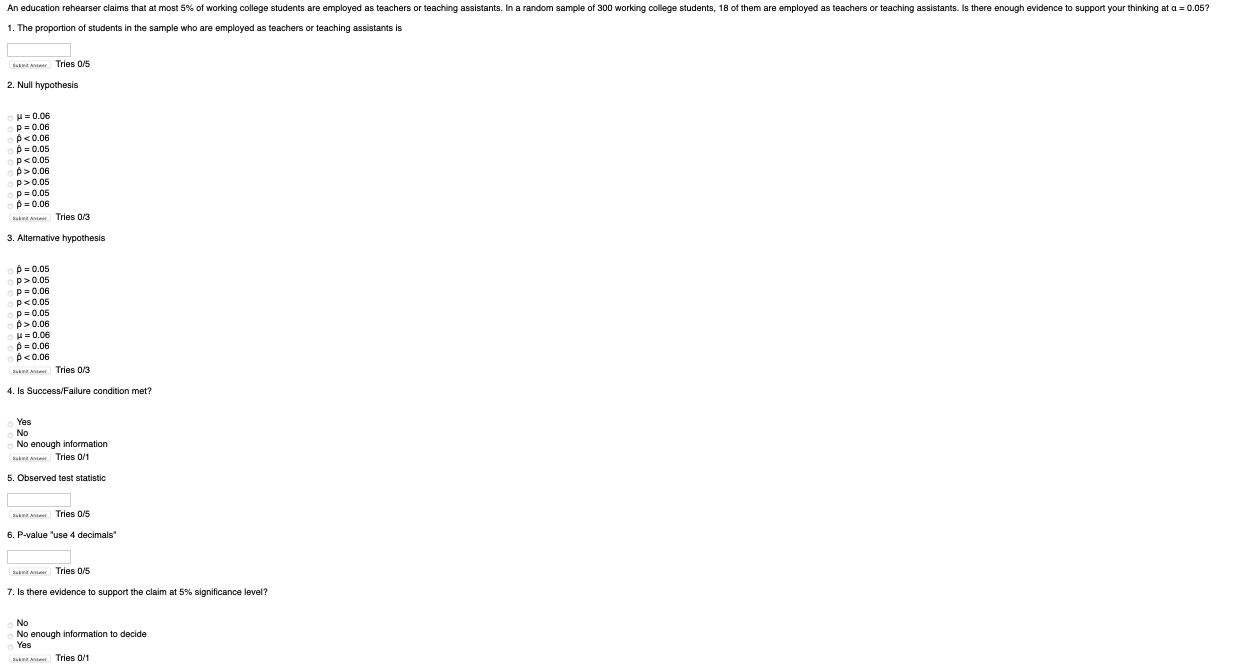The image features a question likely sourced from an exam, presented in small, black text on a plain white background without any bordering. The question centers around an educational hypothesis: an education researcher asserts that no more than 5% of employed college students work as teachers or teaching assistants. In a random sample consisting of 300 working college students, 18 are found to hold such positions. The main task is to determine if there's sufficient evidence to challenge this claim at a significance level of 0.05. 

Below the question, there's an open white response box. Underneath that, in black text, it reads "tries 0 of 5." The subsequent numbered prompts guide the responder through the hypothesis testing process: 

1. "Null hypothesis," accompanied by a selection of potential answers and the note "tries 0 of 3.";
2. "Alternative hypothesis," also followed by multiple choices with "tries 0 of 3.";
3. "Is success/failure condition met?" with options "Yes," "No," and "Not enough information," and "tries 0 of 1.";
4. "Observed test statistic," with "tries 0 of 5.";
5. "P-value," with a note to "use four decimals."

This detailed structure suggests a comprehensive assessment tool aimed to evaluate the student's understanding and application of statistical testing principles in educational research.